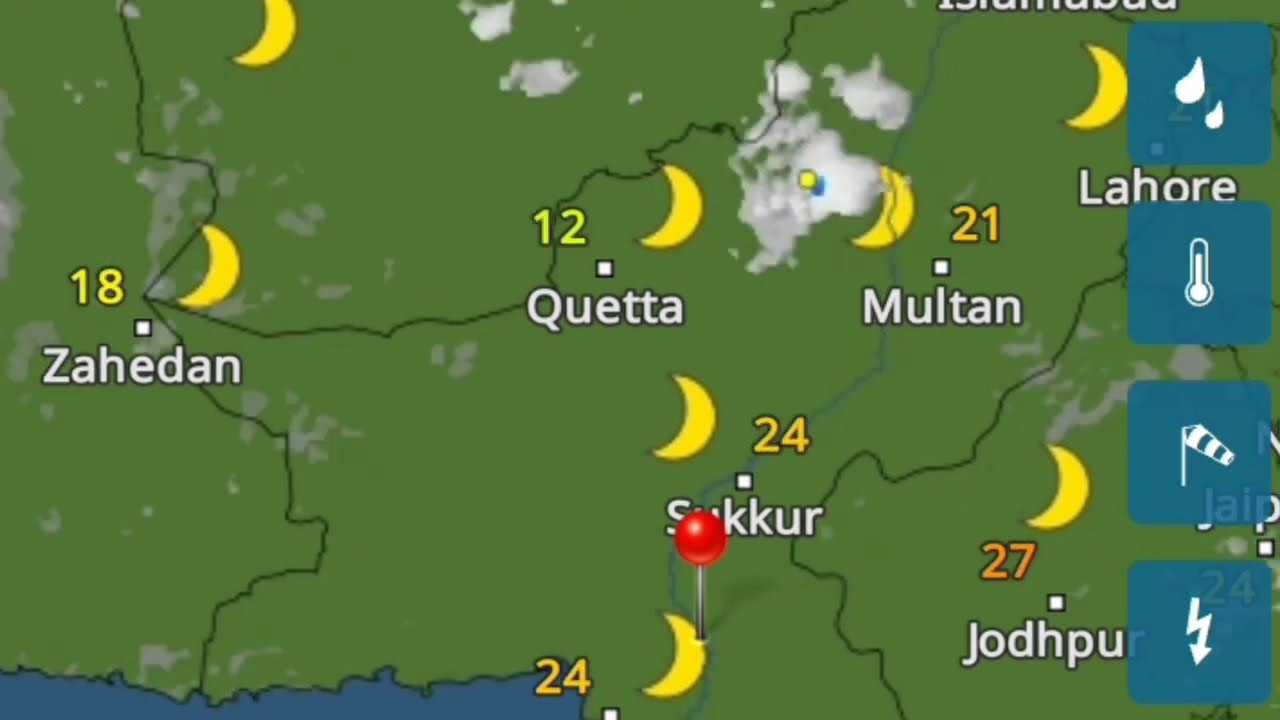The image depicts a detailed weather map similar to those featured on TV weather segments. It showcases a green territory segmented by black lines into different areas, likely indicating countries or states. Over various parts of the map, there are names of cities marked in white, including Zahidan in the west, Quetta in the central area, Multan to its east, Sukkur to the southwest, and Jodhpur to the south.

Each city is accompanied by a crescent moon symbol, suggesting nighttime, and numbers that probably indicate temperatures, such as 12, 24, and 27. Additionally, white cloud graphics float over different regions, hinting at cloudy weather. On the right edge of the map, three semi-transparent blue squares run vertically, each bearing a different white symbol: water droplets for precipitation, a thermometer for temperature, a wind measurement flag for wind speed, and a jagged arrow possibly indicating changes or disturbances. The map layout hints at a comprehensive weather forecast, combining temperature, cloud cover, and other meteorological data for the listed cities.